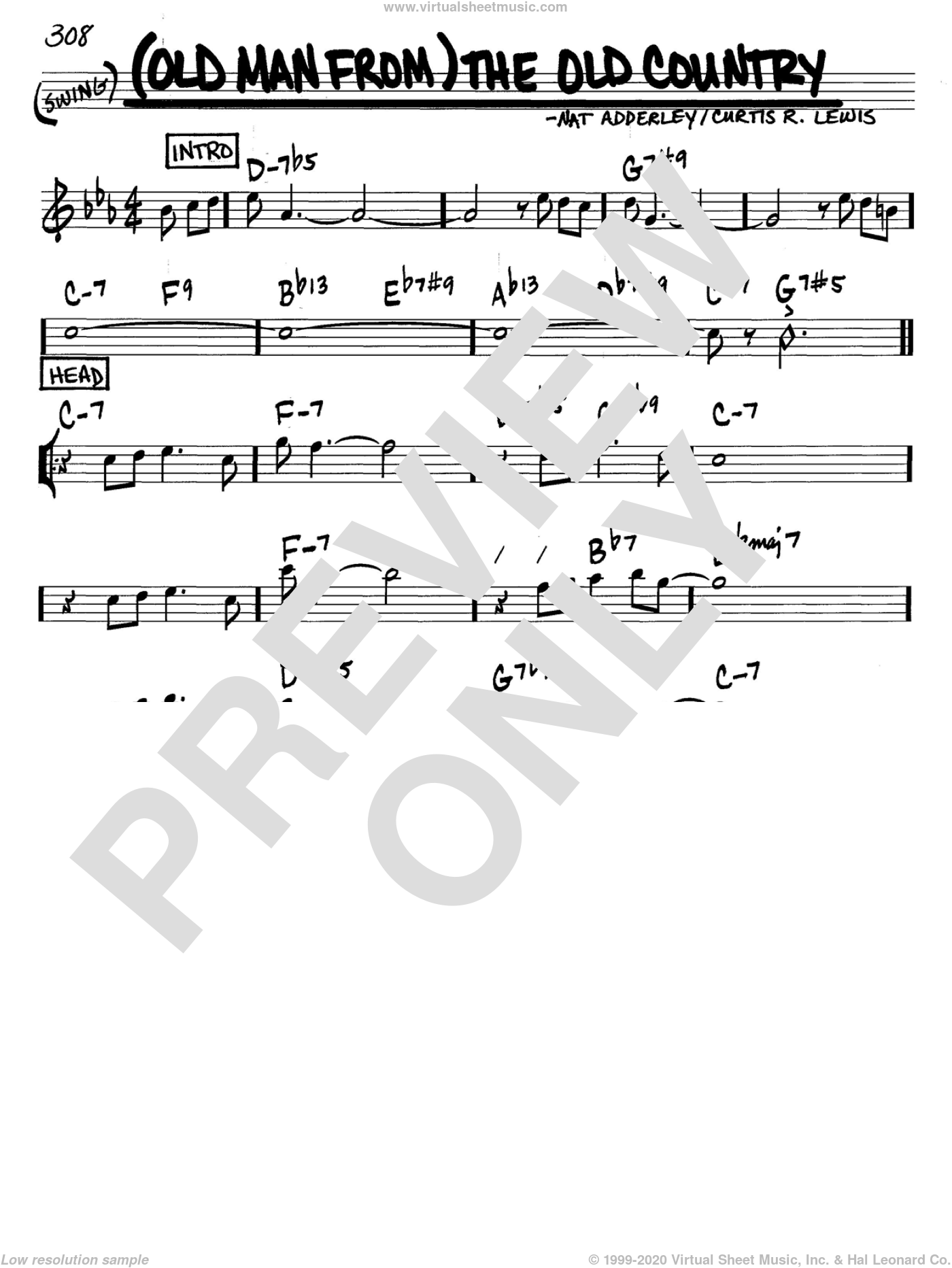The image is a detailed sheet of music for the song "The Old Country" by Nat Adderley and Curtis R. Lewis, available at www.virtualsheetmusic.com. In bold, black handwriting font, the title "Old Man from the Old Country" is prominently displayed with "(Swing)" in parentheses at the very start, and the number "308" in the upper left corner. The entire sheet is monochromatic with the exception of the large gray text "Preview Only" diagonally stamped across the page at a 45-degree angle, indicating it is a preview version. The sheet music features four lines of musical notation, with labels "Intro" and "Head" marking sections of the music. Above and on the scales, various musical notes are displayed. At the bottom, additional text states "Low Resolution Sample, copyright 1999-2020, Virtual Sheet Music Incorporated, and Howe Leonard Company."